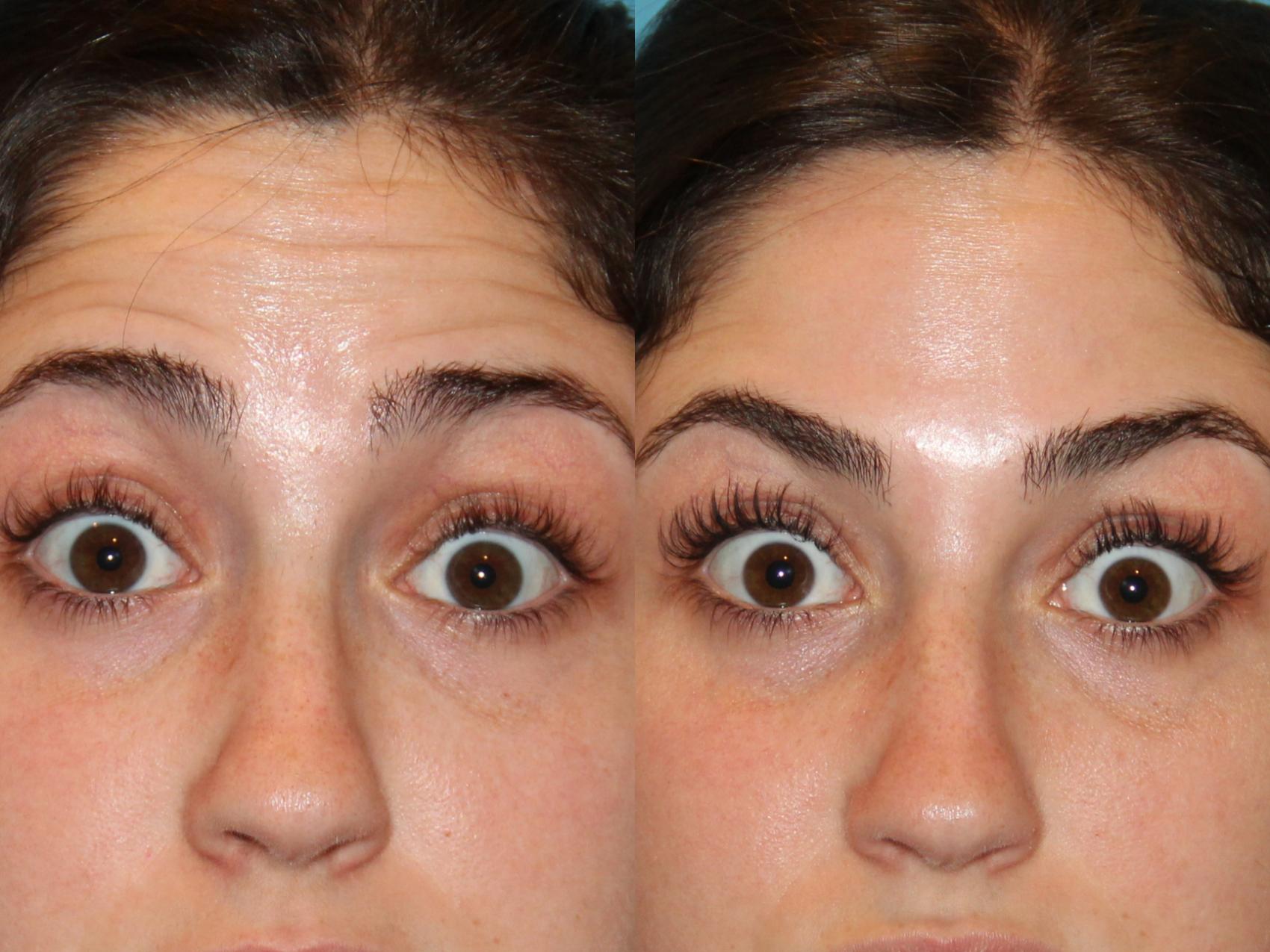The photograph presents a mysterious, double portrait of a Caucasian woman with dark hair and brown eyes, her frames ending where her lips begin. This composite image appears to depict the same woman in two slightly different expressions, possibly manipulated or edited. Both halves show her wide-eyed with raised eyebrows, but the left side features prominent forehead wrinkles suggesting a more surprised expression, while the right side displays a smoother forehead, indicating the effect of a cosmetic procedure. Her dark brown hair, likely pulled back, and her curled eyelashes, possibly enhanced, complete this enigmatic and detailed portrayal. The image captures the subtle yet distinct changes in her facial expressions and skin texture, emphasizing the transformative effect, be it digital or cosmetic.